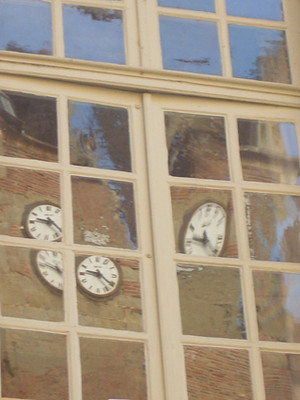This is a detailed color photograph depicting a section of a tall stone building with a vertical arrangement of windows. The structure includes both doorways and paned windows with off-white frames and mullions. The window panes are separated by brown wood and appear to consist of multiple small squares within a larger frame. Reflected in the warped glass panes are four white clock faces with black hands, possibly part of the iconic Big Ben, set against the building’s stone facade. The clocks' reflections are distorted slightly, showing their numbers clearly though specific finer details of the stonework are less discernible. The sky, which is clear and blue, is also faintly reflected at the top of the windows. This scene is captured from a slightly upward angle, making the image taller than it is wide. The building material appears to be a reddish-brown stone, contributing to the warm tones of the photograph. There are no people, plants, animals, signs, or vehicles in this image, emphasizing the architectural elements and their reflections.